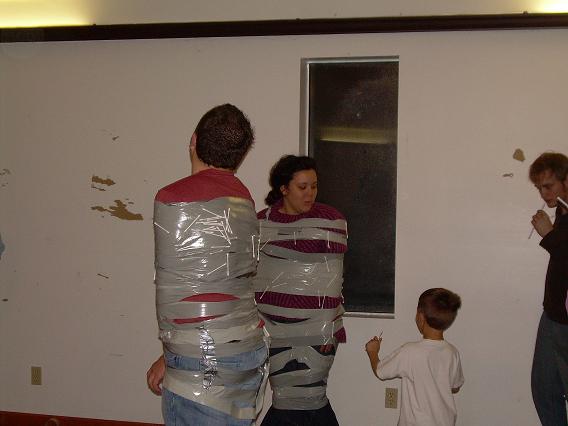In this intriguing and somewhat humorous photograph, we observe two adults, a man and a woman, who are tightly bound with a mixture of grey industrial tape and small white items, possibly Q-tips. Both are attired in red shirts and denim bottoms. The man, with short brown hair, faces the wall while the woman with fuzzy black hair looks down at a young boy, who is standing beside them. This boy, likely around the same height as a small window in the background, has short brown hair and wears a white short-sleeved shirt. The scene suggests a playful setting, potentially involving the child and adults in a game. Another man, positioned to the right, leans towards the boy with a straw-like object pointed at his mouth. This individual dons a dark long-sleeved shirt and grey pants. The backdrop features a chipped white wall revealing brown patches, a black window, and a ceiling with a strip of dark brown wood, consolidating the environment as a worn but cozy room. The entire setup hints at a spirited family moment or a playful challenge in progress.